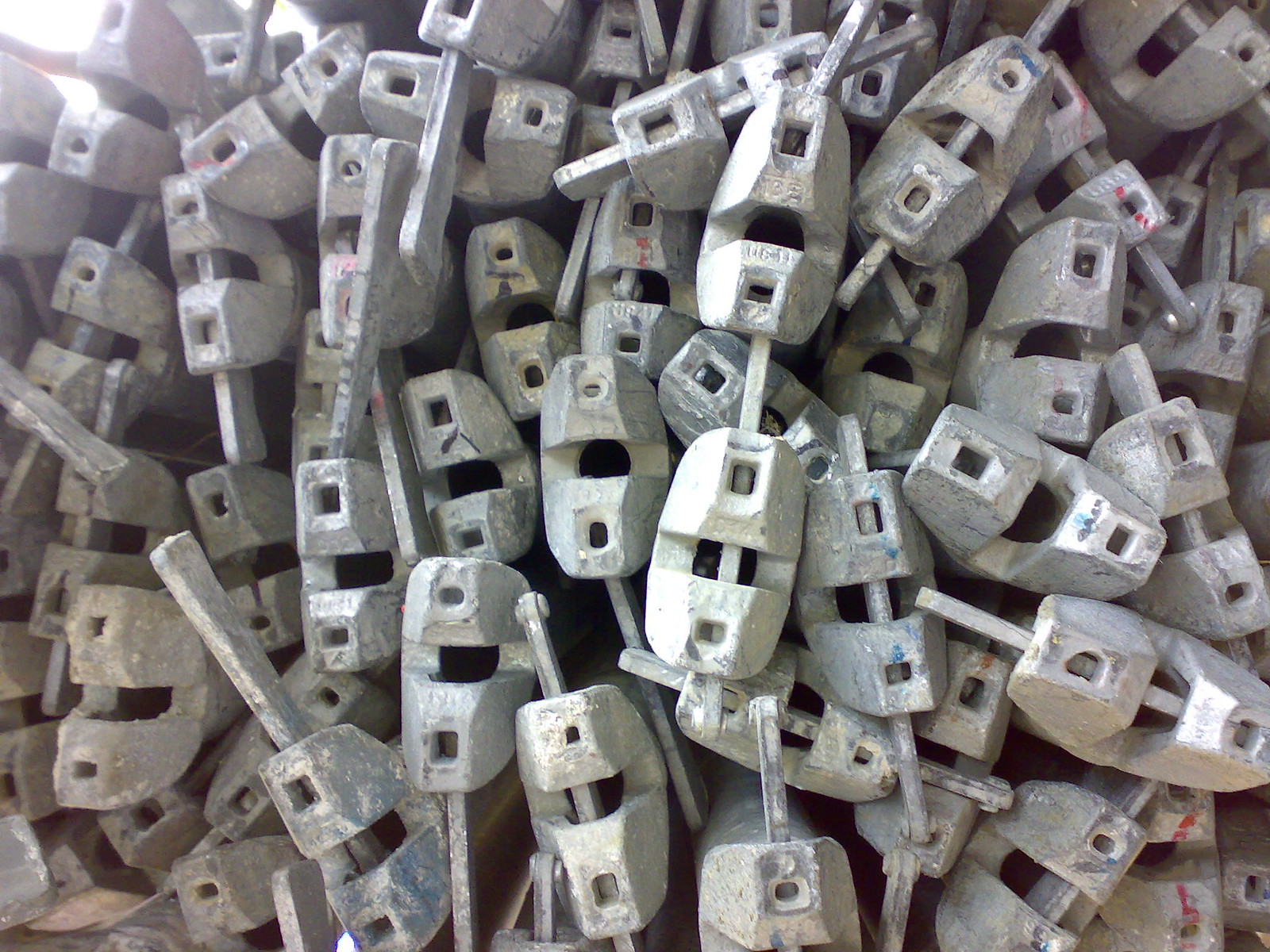The photograph depicts a significant number of uniformly shaped metallic devices, stacked closely together in a well-lit area. Each device is primarily light gray in color, though some exhibit smudges of red or blue. They share a roughly rectangular, hollow structure with three holes—two near the vertical top and bottom, and one centrally placed. An elongated rod extends vertically through each device, resembling a handle or connector. The metal appears somewhat corroded in places, giving a textured, stone-like appearance. The devices are packed so tightly that they maintain a straight, upright position, and they dominate the entire image, with no other elements visible.